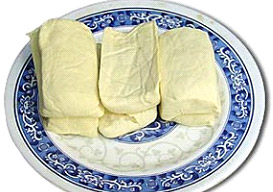This image features a detailed blue and white plate with intricate designs. The plate's design starts with a white outer edge, followed by a blue ring, a narrow blue pinstripe, another white ring, and a blue center adorned with white decorative scrolls, giving it an elegant, China-like appearance. Positioned on the plate are six food items, evenly laid out in two rows of three. These items are white and resemble tightly rolled flatbreads, possibly tortillas filled with an unknown ingredient and folded to form horizontal rectangular shapes. The background of the image is simple and white, emphasizing the plate and its contents.